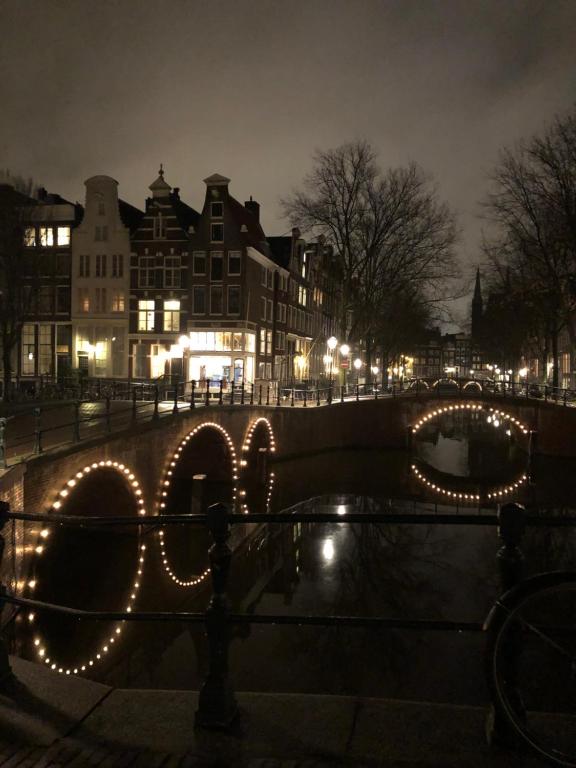This full-color photograph captures a picturesque night scene from a bridge overlooking a canal in a charming town. The image, taken vertically without a border, showcases the soft glow of artificial lights illuminating the scene. The night sky is overcast with gray clouds, faintly glowing with distant lights. 

In the foreground, there's a low-hanging bridge with an arch, adorned with bright whitish-yellow and amber-colored lights that drape over the archway, reflecting beautifully on the water below. Further up the canal, another bridge with three arches continues the theme, also festooned with similar lights. 

To the right of the image, tall, bare trees without leaves create a stark silhouette against the lit scene. On the left, buildings made of brick, approximately four to five stories high, line the street. These structures have a distinctive triangular upper story design and are warmly lit with street lamps and interior lights, hinting at bustling storefronts along the ground level. The street and buildings give a cozy, bustling impression despite the late hour, with a row of street lamps adding to the serene ambiance.